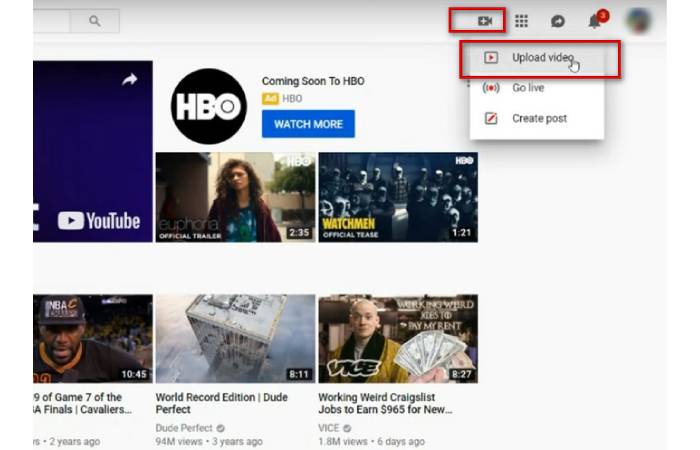The image is a screenshot of a YouTube interface. On the right side of the screen, there are a few icons, starting with a camera icon highlighted by a red rectangle. A drop-down menu below the camera icon shows three options. The first option, also highlighted with the same red rectangle, reads "Upload video." The second option, outside of the highlighted area, says "Go live," and the last option reads "Create post."

On the left side of the screen, there is an advertisement for HBO. The ad text states "Coming soon to HBO," and is accompanied by the HBO logo. Below the logo, there is a button labeled "Add HBO," and next to it, a blue button that says "Watch more." Additionally, there are several video thumbnails displayed, which appear to be trailers.

This descriptive caption provides a detailed overview of the elements present in the YouTube screenshot, giving a clear understanding of the content and options shown in the image.